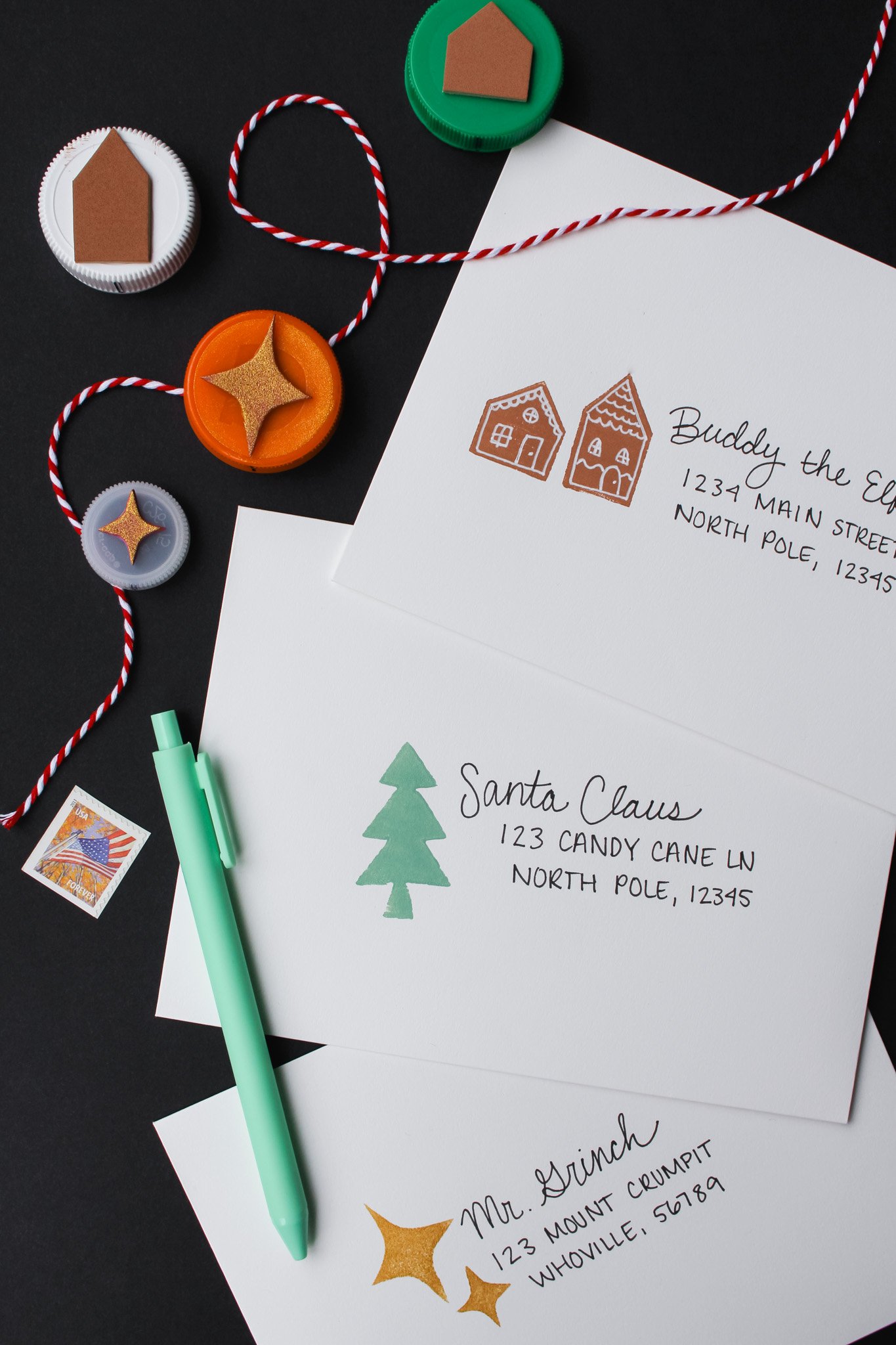Against a solid black background, the photo features three white envelopes with distinct, festive addresses, and various decorative objects. The top envelope, displaying two brown gingerbread houses of different sizes, is addressed to "Buddy the Elf, 1234 Main Street, North Pole, 12345." The middle envelope, with a green Christmas tree made of three stacked triangles and a base, reads "Santa Claus, 123 Candy Cane Lane, North Pole, 12345." The bottom envelope, adorned with two gold four-pointed stars, is addressed to "Mr. Grinch, 123 Mount Crumpet, Whoville, 56789." A seafoam green pen lies diagonally across the envelopes, and to the left, there is a stamp featuring the American flag, a piece of red and white string, and green, orange, and white bottle caps decorated with images of homes and stars.